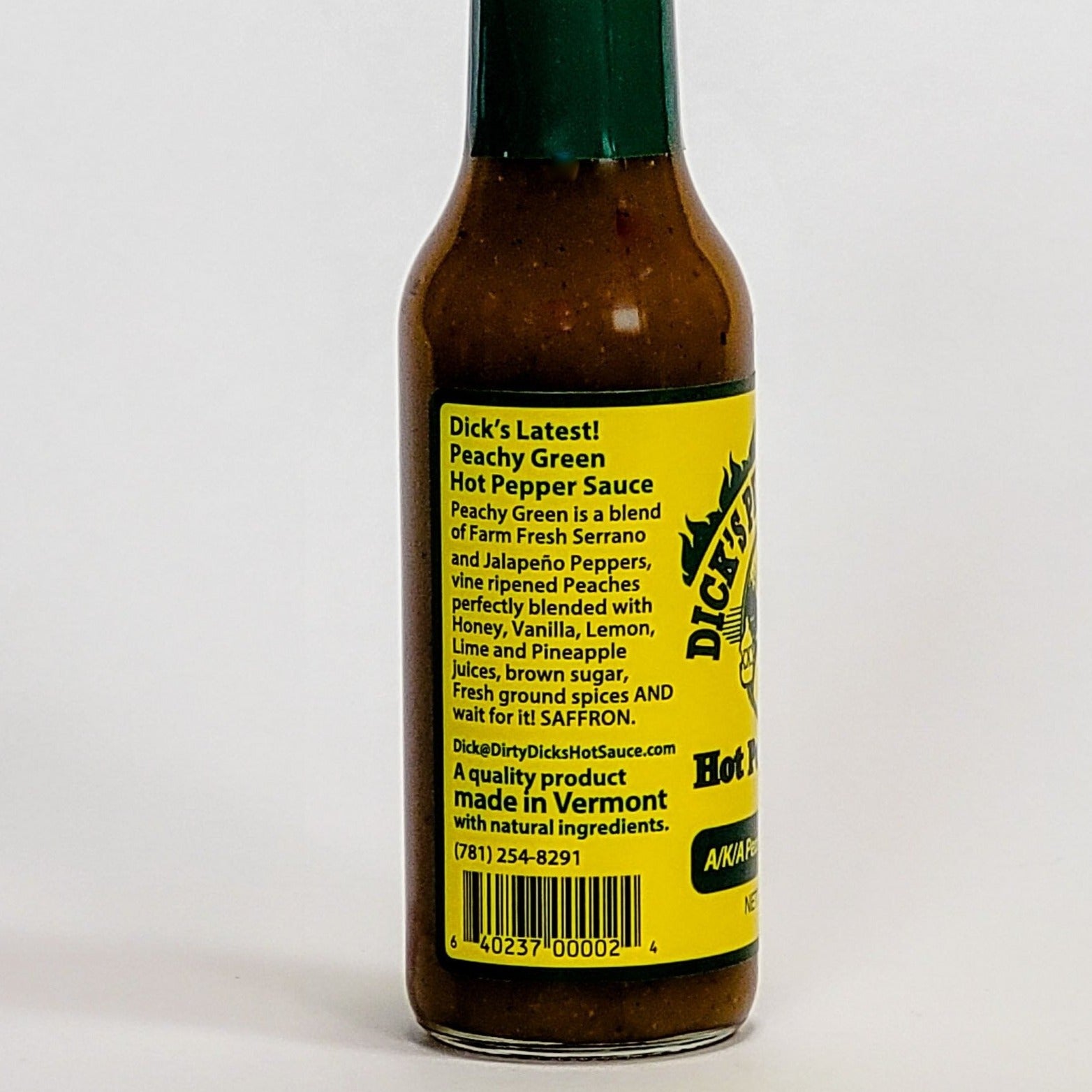The image depicts a bottle of Dick's Latest Peachy Green Hot Pepper Sauce, prominently featuring a vibrant yellow label with black text. This bottle, with a sealed tear-off top, showcases visible seeds suspended within the reddish-brown liquid inside. The label details the sauce as a blend of farm-fresh serrano and jalapeno peppers, vine-ripened peaches, honey, vanilla, lemon, lime, and pineapple juices, supplemented with brown sugar, freshly ground spices, and saffron. 

At the top of the label, in bold letters, it reads "Dick's Latest Peachy Green Hot Pepper Sauce." The bottom of the label includes a UPC barcode and the contact details which specify the product's Vermont origin and a contact email: dick@dirtydickshotsauce.com, complemented by the number 781-254-8291. The bottle itself stands against a white background, emphasizing its detailed label and content.